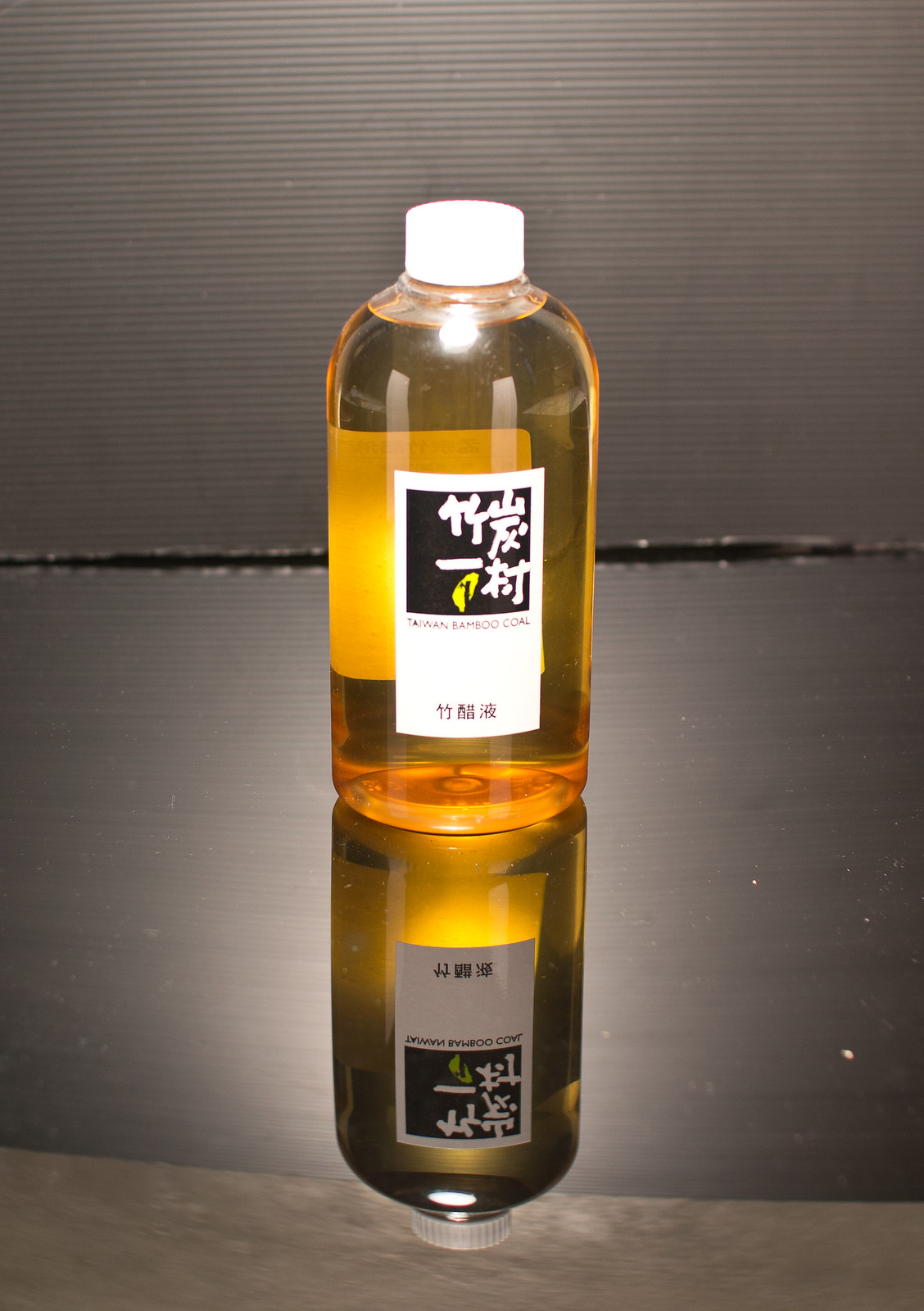The photograph captures a clear, rectangular plastic bottle with rounded edges, filled with an amber-colored liquid. The bottle features a white twist cap and a white label on the front, which includes a black rectangle with several Asian characters, followed by the text "Taiwan Bamboo Coal." The bottle is positioned on a black, highly reflective surface, creating a mirrored image directly below it. The backdrop consists of black, ridged plastic material with subtle lighting highlighting its texture. Through the transparent bottle, the back of the front label and an additional white label on the back are visible, though the exact text is obscured.